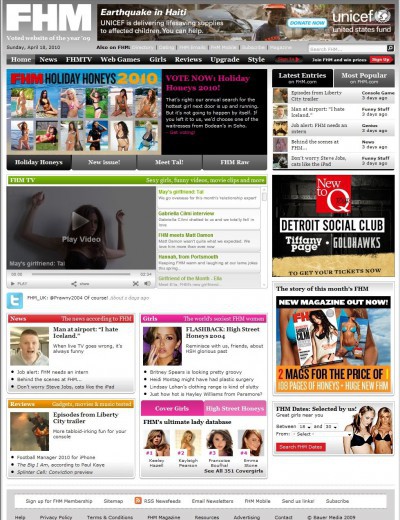The image appears to be a screenshot from a website dating back to approximately 2010. In the upper right corner, there is a prominent UNICEF advertisement related to the earthquake in Haiti, featuring an appeal for donations to support life-saving supplies for children affected by the disaster. The advertisement includes the UNICEF logo, and a "Donate Now" button, set against a backdrop of devastation with an African child wearing an orange hat amidst wreckage, including a damaged car. Just below the ad, the text indicates "Limited States Fund" or a similar message.

In the upper left corner of the image, in small print, the date "Sunday, April 28th, 2010" is faintly visible. Above this date, bold white letters spell out "FHM" against a gray background. To the right of the date are various clickable options, although the text is too small to read. On the far right, there's a search bar.

The midsection of the webpage is densely packed with content. One notable element is a video thumbnail featuring a Caucasian woman with shoulder-length hair and her arms raised, with a "Play Video" button and the ambiguous text "Mae's Girlfriend, Ty" at the bottom left of this thumbnail. Below this, a section labeled "News" in a prominent red bar displays a picture of a short Caucasian man with brown hair wearing a gray shirt. The caption under the image, though partially obscured, seems to read "man at airport, I hate Iceland." Three additional articles are listed below this image.

At the bottom of the page, a gold bar labeled "Reviews" in white text is partially readable, indicating this might be a section dedicated to reviews. Below this bar, there is an image from what appears to be a movie, showing a man holding a source of light, accompanied by the title "explode episodes from Liberty City trailer" and three more options to explore.

In the upper right part of the image, there is a pink box with the word "Girls" in white letters, followed by an unreadable text. Adjacent to this is a picture of a Caucasian woman with her hand beside her face and the caption "flashback, high street, honey's 2004," along with four clickable options underneath. The term "high street" is a giveaway that this website is likely UK-based, as it is a common term used for main streets in the UK.

Overall, the webpage is cluttered with numerous advertisements and articles, pointing towards a women's magazine website from the UK, with a design and content style typical of the early 2010s.